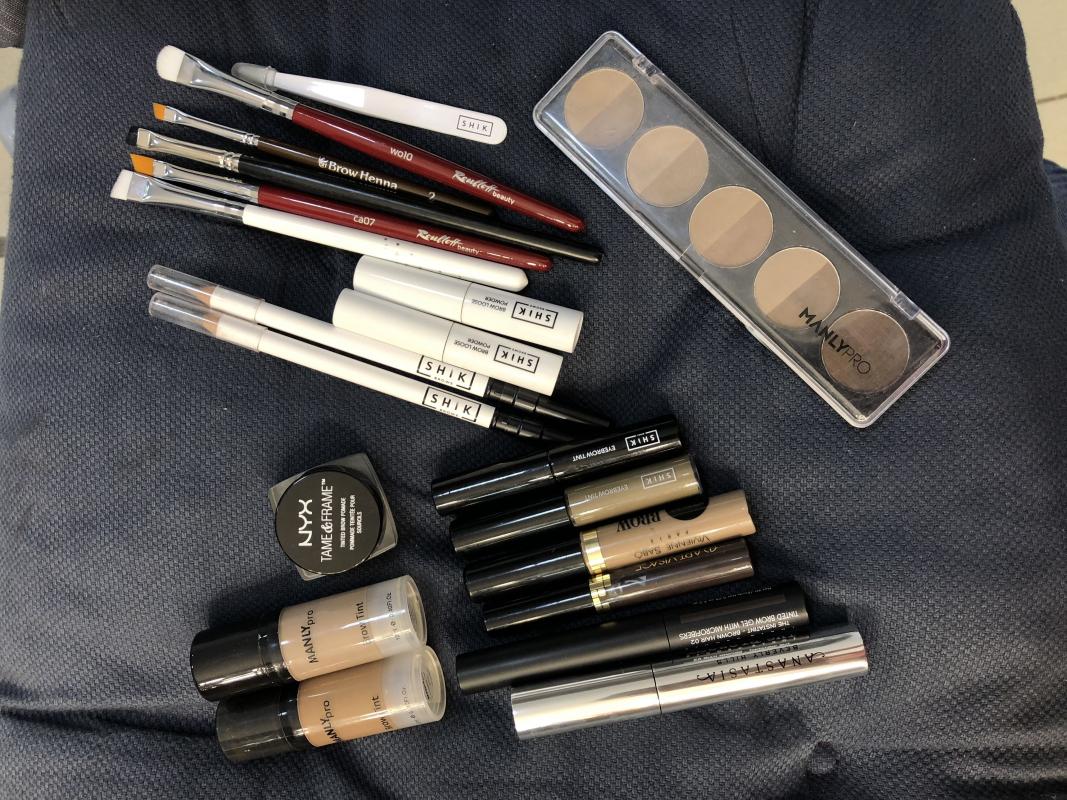The image showcases an array of cosmetics and cosmetic accessories meticulously arranged on a textured, black-cushioned surface adorned with black buttons. In the background, a beige shade occupies the top right corner, while an indistinct object is partially visible on the left. 

At the top of the arrangement, there is a collection of small, angled makeup brushes, including a white tweezer, a red brush, a black brush, a brown brush, another red brush, and a white brush. Below these brushes, there are two lip balms and what appear to be two colored eye pencils. 

Further down, the display includes an assortment of foundations, mascaras, and a small black tube containing primer. A color palette designed for shading is also present, featuring four distinct shades split in half, with a darker tone positioned on the far right. 

The makeup brands visible in the image include "Chic" and "NYX," while some other labels are not legible.